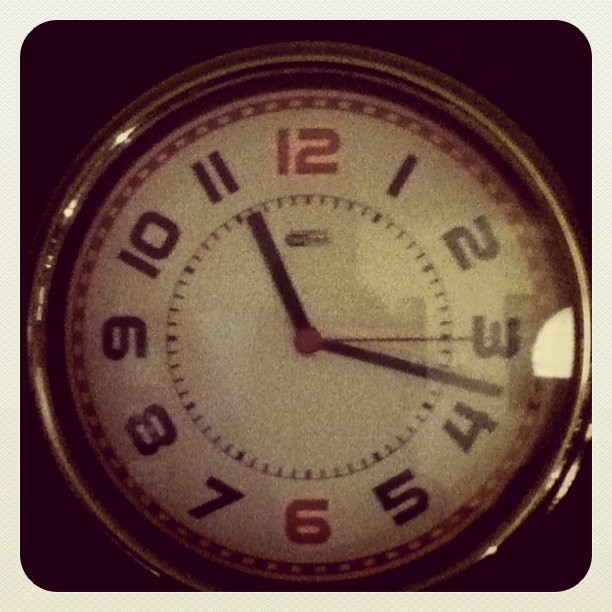The image in question is a grainy, square photograph with rounded edges and a white border, possibly resembling an Instagram-style post. Featured centrally is an antique-looking clock with a metallic light gold or silver frame. The clock has a distinct design on the face: an outer black border, followed by a white border, and an inner dashed red border. The clock's numbers are a mix of black and red, with the 12 and 6 in red, and all other numbers in black. The minute and hour hands are positioned at approximately 11 and 18 minutes past the hour, respectively, while the second hand points to 15 seconds. The hands are black and red, matching the center mechanism. Notably, the clock has markings for the minutes around its face, enhancing its precision. The glass cover of the clock appears slightly concave, casting a reflection that includes a light source and a faint outline of the person taking the photo. The overall aesthetic and details suggest an old-fashioned or vintage design. The background of the photo is black, adding to the image’s contrasting elements.